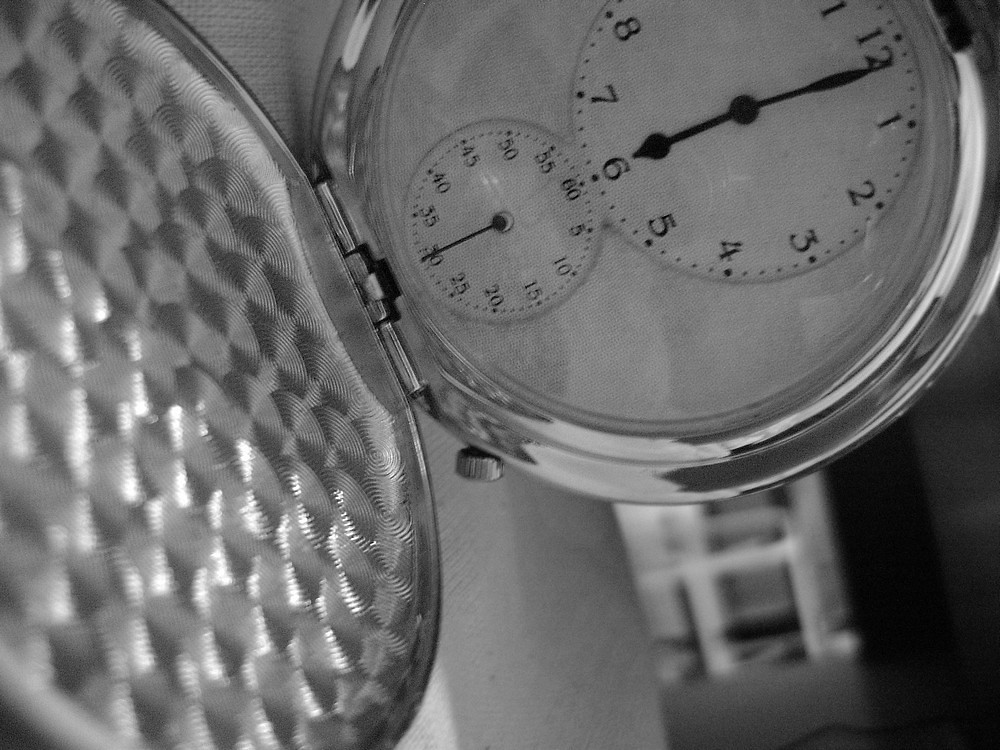The black and white photograph provides a detailed close-up view of an ornate silver pocket watch. The image is rotated 90 degrees to the right, revealing the pocket watch's interior with its open cover resting on the ground. The main clock face, positioned in the top-right portion of the photo, displays the time as just after 6:00 with black numbers from 1 to 12 and corresponding minute markings. Beneath the main dial is a smaller, intricate seconds dial marked by numbers in 5-second increments, starting from 60 at the top. The subtle silver background seen behind the slightly tilted pocket watch adds to the overall vintage aesthetic, while the rest of the frame vaguely hints at an indistinct room setting.